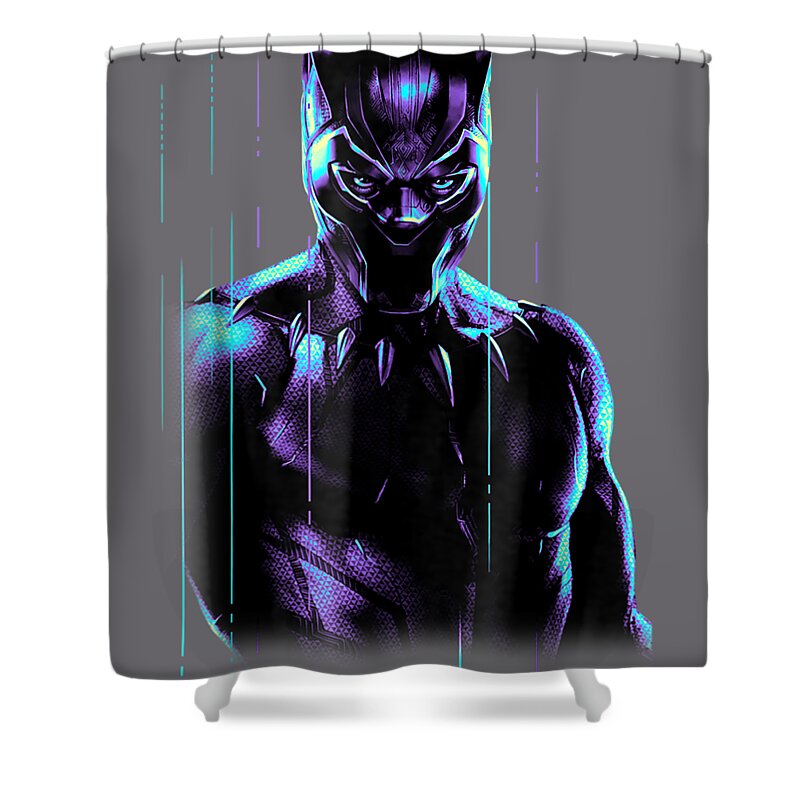This is an image of a shower curtain hanging on an arced rod around a pedestal tub, of which only the feet are visible. The curtain features a detailed depiction of Black Panther, a comic book character from Marvel. Black Panther has a purplish-blue tint, muscular appearance, and wears a sleek suit that highlights his powerful physique. His mask covers his face except for his striking blue eyes, which peer directly at the viewer. Notably, light blue and light purple streaks overlay parts of the character, adding a dynamic, almost electrical effect to the scene. The background of the curtain is a medium gray, enhancing the starkness of Black Panther's image. The overall setting gives a somewhat dark and intense atmosphere, elevating the dramatic visual impact of the curtain.